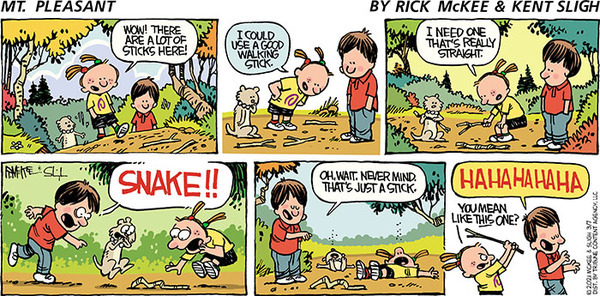This detailed image frame from the vibrant and colorful comic "Mount Pleasant" by Rick McGee and Kent Sly provides an amusing snippet of a forest adventure involving two children and a small animal. The comic is laid out in six distinct panels. In the first panel, a child with pigtails and another child in a red shirt walk through a forest, accompanied by what seems to be a small animal. The pigtail child remarks on the abundance of sticks. The second panel shows them considering the need for a good walking stick as they look down at the ground cluttered with sticks. The third panel has the pigtail child, now bending down, seeking a particularly straight stick.

In the fourth panel, the child suddenly exclaims, "Snake!" alarming everyone as the supposed walking stick writhes. However, in the fifth panel, the child in the red shirt corrects the alarm, realizing it's just a stick. Both the pigtail child and the small animal are shown collapsed in mock fear or exhaustion. The final panel adds a twist of humor with the pigtail child standing behind the red-shirted child holding a stick, hinting at playful revenge for the false alarm. The red-shirted child laughs, while the pigtail child prepares to whack him, adding a layer of playful interaction and camaraderie to their forest tale.